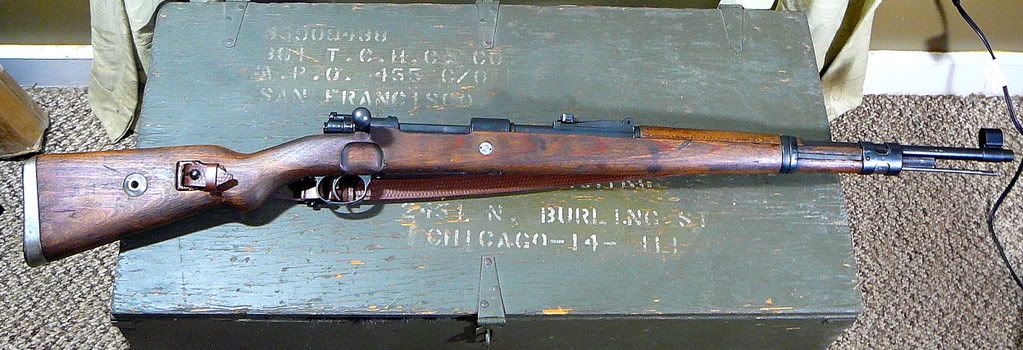The image showcases an antique-style rifle with a wooden brown stock and black metal components, including the barrel and trigger. The rifle lies horizontally, facing right, atop an aged wooden container that has been painted an olive green but is chipping to reveal yellow wood beneath. The container, which has a central latch, displays faded white stamped letters, including partially visible words like "San Francisco" and "North Burling Street, Chicago." This container rests on a Berber carpeted floor in a light coffee brown shade. In the right side of the image, a cord emerges from a dark brown wall with white baseboards. To the left, the leg of a table is visible, and the upper left corner shows a light gray garment or rag hanging from the backside of the container.